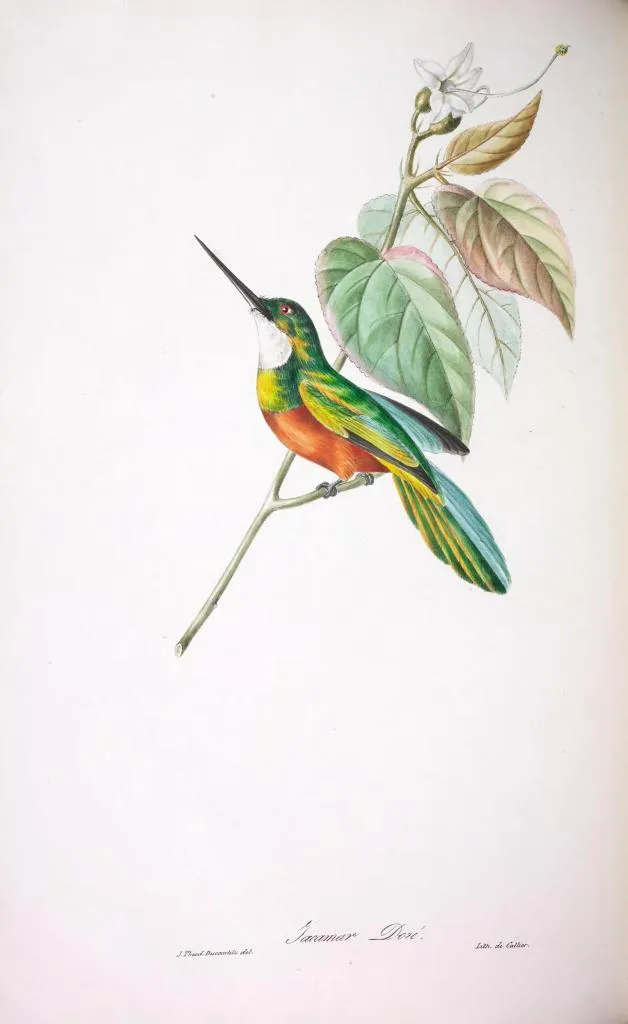This image is a detailed and realistic drawing of a bird perched on a thin, light green branch against an off-white background. The bird is predominantly green and yellow with a reddish-brown stomach and a white patch under its neck. It features dark eyes with hints of red or orange, and a long, sharp black beak. The bird's wings are folded inwards, displaying touches of teal and blue on the feathers. Its tail is a mix of green, yellow, and blue. The branch, seemingly unattached to any tree, supports the bird on its right smaller offshoot, while the left branch extends behind with six leaves in varying shades of green and hints of brown. Additionally, a delicate white flower with white petals and a distinctive white stripe is situated near the top of the branch. The background has a light gray hue, darker at the corners and brighter in the center, enhancing the bird's vivid colors. At the bottom of the image, there is cursive writing, which appears to be a signature or names, but the text is difficult to decipher.